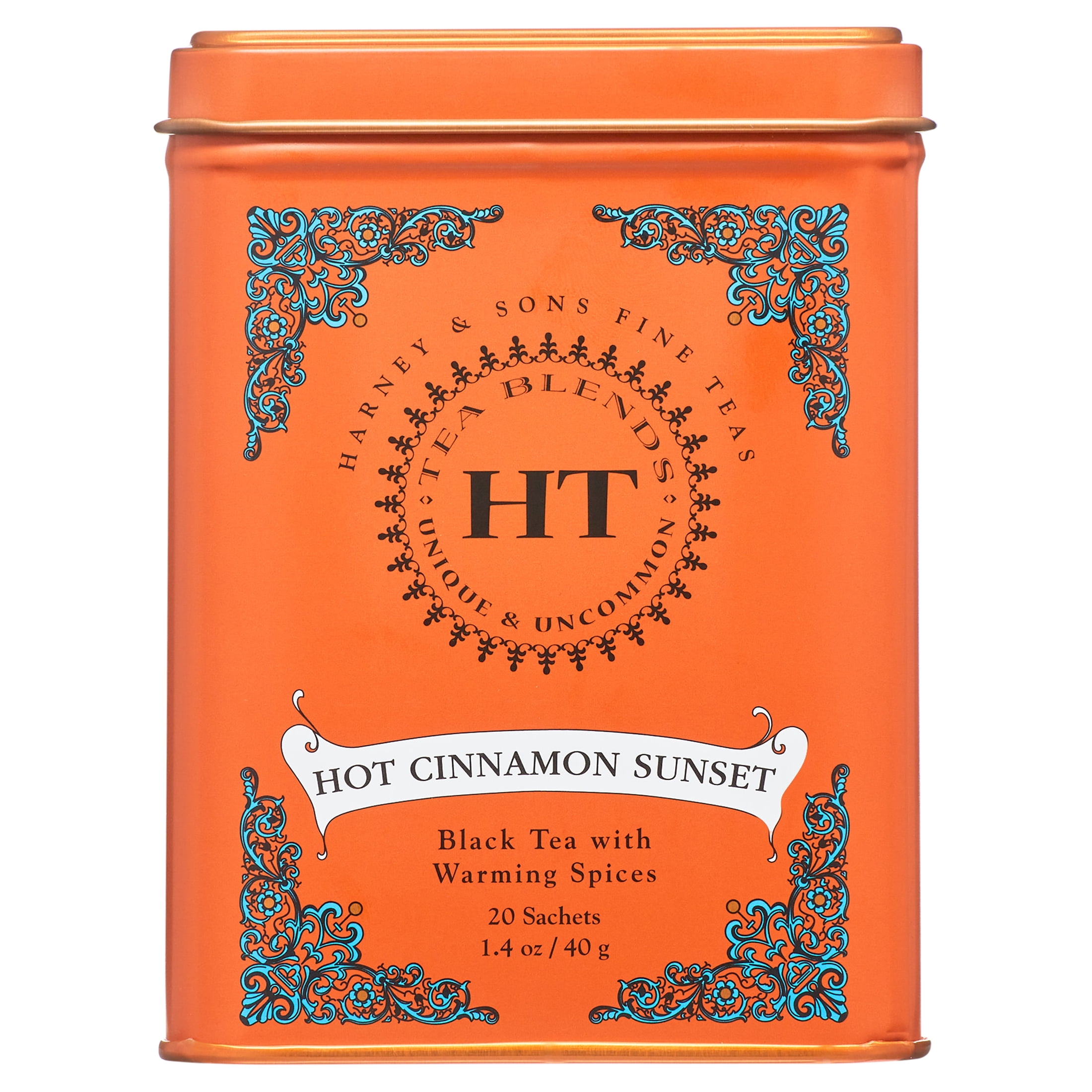The image showcases a high-resolution photograph of a vibrant, warm orange metal tin, specifically designed for tea. The tin appears square and has a lid adorned with a narrow bronze bead around its circumference. The front face is richly detailed with four blue triangular swirly designs at each corner, incorporating intricate flower patterns and resembling mandalas. 

The tin prominently features the logo "HT" in black at its center, likely representing Harney and Sons. Above the logo, an arc of text reads "Harney and Sons Fine Teas," positioned between the top two blue triangles. A circular geometric pattern surrounds the "HT" logo, with the words "Tea Blends" written along the top arc, followed by "Unique and Uncommon" along the bottom arc, separated by dots.

In the lower third section of the tin, a white banner displays in black text "Hot Cinnamon Sunset." Beneath this banner, more black text identifies the product as "Black Tea with Warming Spices," followed by "20 sachets," and lastly, "1.4 OZ / 40G" on the bottom line. The bottom base of the tin also features a thin bronze bezel similar to the lid, giving it a cohesive and old-fashioned yet potentially modern appearance.